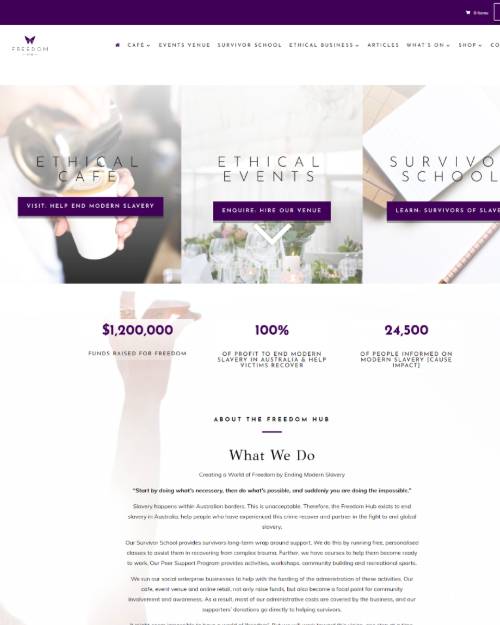**Caption:**

"Freedom Fund is an Australian charity organization dedicated to combating modern-day slavery. Their multifaceted approach includes initiatives such as ethical cafés, events to raise awareness, and survival schools designed to help victims recover. The organization has successfully raised over $1.2 million to support their mission. Freedom Fund educates the public on the critical issue of modern slavery, impacting over 24,500 informed individuals. Their efforts are critical in regions where exploitation is rife, including various parts of the Middle East. Despite the challenges of slavery still existing globally, Freedom Fund's work highlights the importance of international recognition and support in fighting this human rights violation."